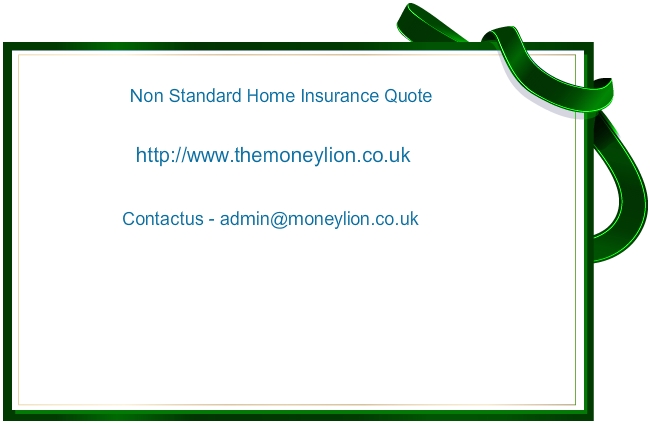The image features a sizable rectangular cardstock, approximately 6 inches wide by 4.5 inches tall, with a distinct green border and a loosely draped green ribbon around the upper right-hand corner. Set against a clean white background, the card prominently displays text in blue print. The top line reads "NON-STANDARD HOME INSURANCE QUOTE". Below that, in smaller text, it reads "http://www.themoneyline.co.uk" and "Contact us at admin@moneyline.co.uk". The image appears to be web-generated, likely using a pre-made template, conveying essential information simply and clearly without any additional graphics or elements.